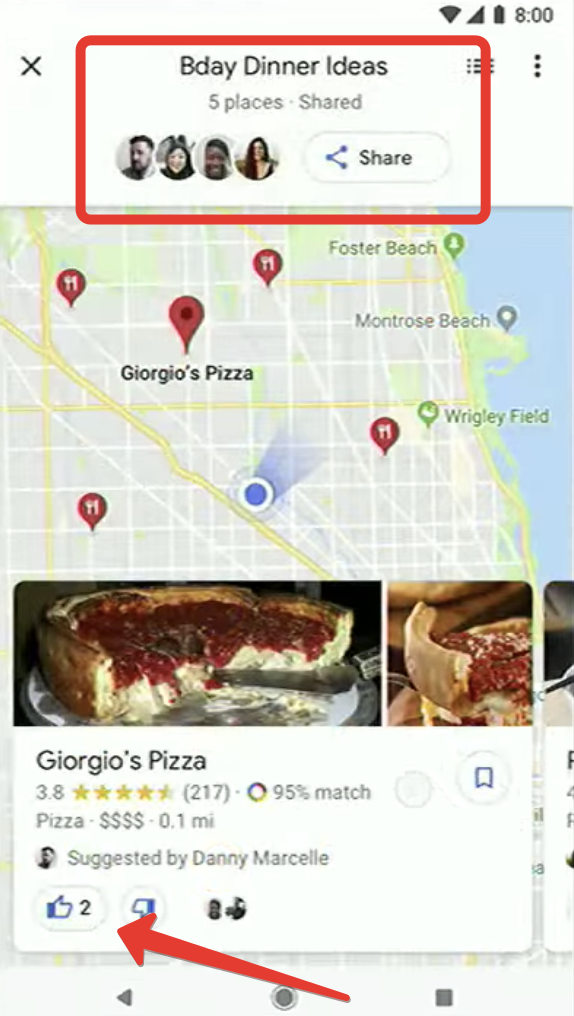The image depicts a Google Maps screenshot featuring a shared list titled "B-Day Dinner Ideas." Within this list, there are five places suggested, though only one is visible: Giorgio's Pizza. The name Giorgio's Pizza is spelled out and prominently displayed. This restaurant has garnered two likes, evident from the like and dislike buttons at the bottom of its entry. Currently, Giorgio's Pizza holds a 3.8-star rating based on 217 reviews and is classified as a high-end establishment, indicated by four dollar signs ($$$$). The restaurant is a short distance from the user, precisely 0.1 mile away. The list can be shared with others, as highlighted by a share button and icons of the people with whom the list is shared, all encapsulated within a rectangular border at the top of the screen.